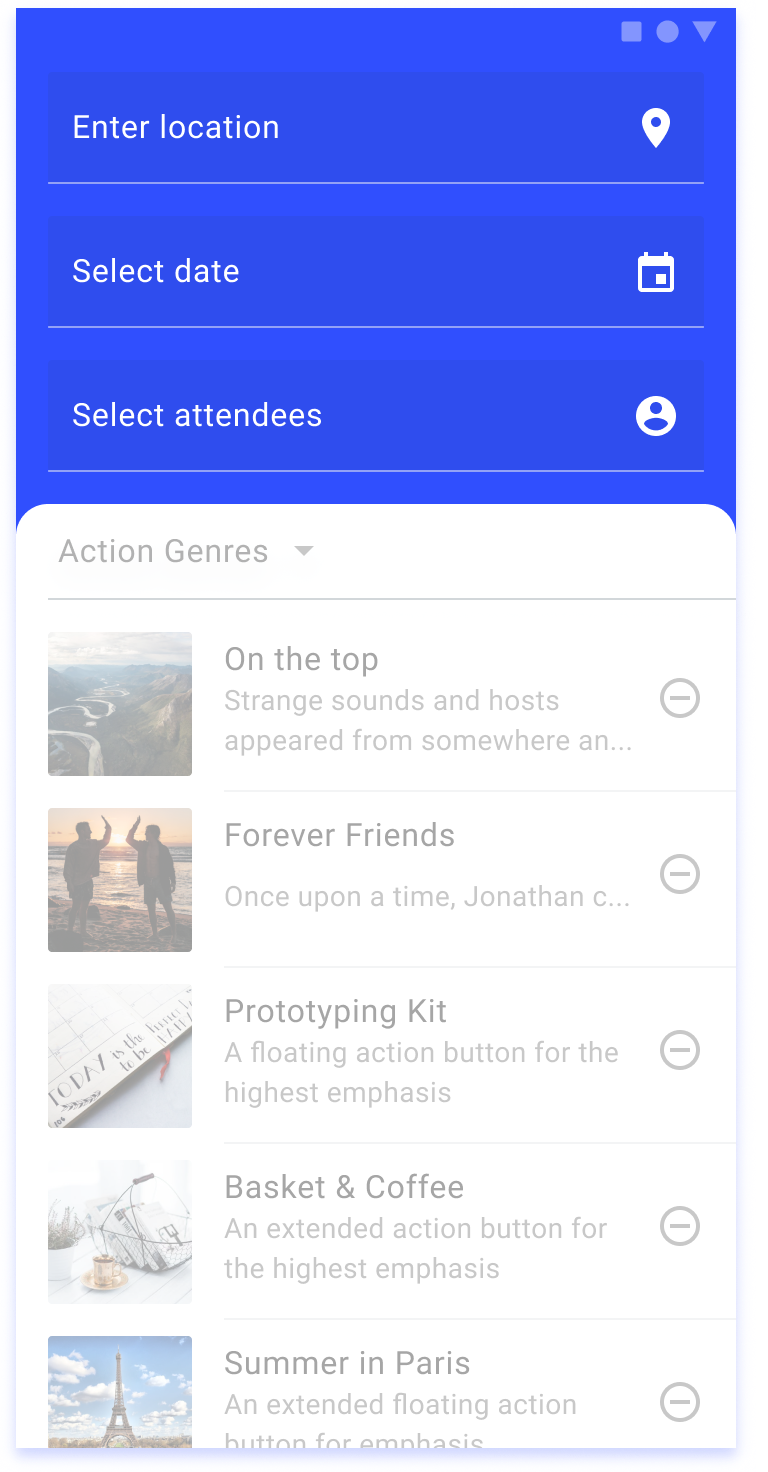This colored screenshot captures the interface of an unidentified application. At the very top, set against a blue background, are three options: "Enter Location," "Select Date," and "Select Attendees." Below this, a slightly faded white section displays the heading "Action Genres." 

Listed within this section are various text entries:
- "Strange Sounds and Hosts Appear From Somewhere and ... Forever Friends"
- "Once Upon a Time, Jonathan C ..."
- "Prototyping Kit, a Floating Action Button for the Highest Emphasis"
- "Basket and Coffee, an Extended Action Button for the Highest Emphasis"
- "Summer in Paris, an Extended Floating Action Button for Emphasis"

Accompanying these texts are a series of vertically formatted, faded photographs:
1. The top photo shows an aerial view of a mountain range with a long, winding white path in the center.
2. The next image captures two individuals about to high-five on a beach at sunset.
3. A calendar page featuring an inspirational saying, although only the word "Today" is discernible.
4. An image of a wire basket filled with various items.
5. A small gold teacup on a matching saucer alongside a potted plant in a white pot.
6. The final photo showcases the Eiffel Tower set against a blue, cloudy sky.

The images provide a varied and visually rich representation, enhancing the textual elements of the app interface.